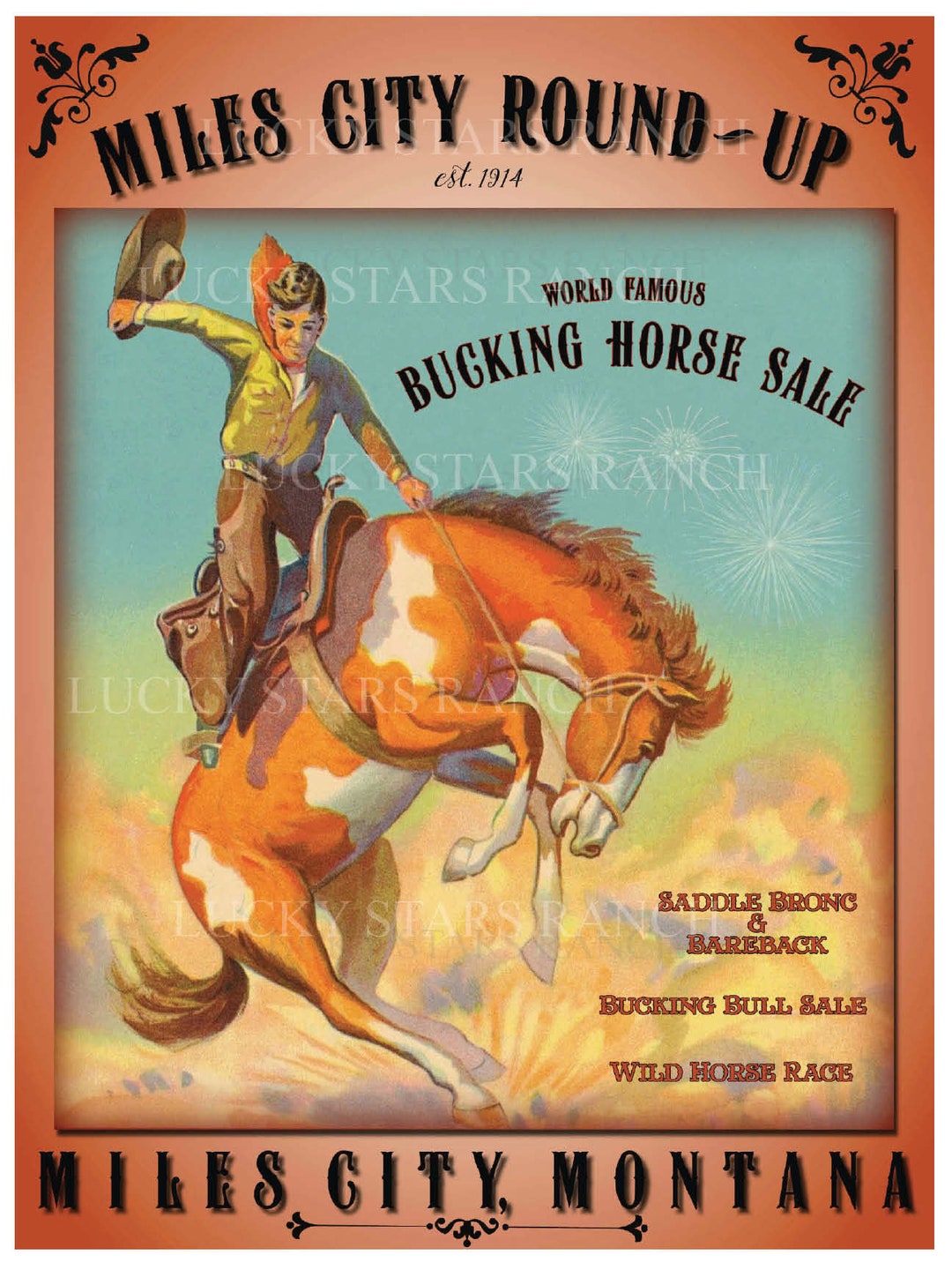The poster, designed with a gradient orangey-red background, serves as an advertisement that you might find in a city or county magazine or even a newspaper. At the top, bold black letters proclaim "Miles City Roundup," with "Established 1914" in a smaller, cursive style beneath. Central to the poster is an illustration, possibly rendered in acrylic paint, of a young cowboy riding a bucking horse. The cowboy, wearing a yellow shirt, brown cowboy pants, and a kerchief fluttering around his neck, grips the reins with one hand while holding his hat high with the other. The horse, depicted in vibrant shades of orange and white with a brown mane, is captured mid-buck with its hind legs in the air and head down. To the right of this dynamic scene, text in white declares "World Famous Bucking Horse Sale." Further down, still on the right, orange letters detail the events: "Saddle Bronc, Bareback Bucking Bull Sale, Wild Horse Race." At the bottom, "Miles City, Montana" is written in black against the orange backdrop, completing the vintage and lively design of this historic poster.